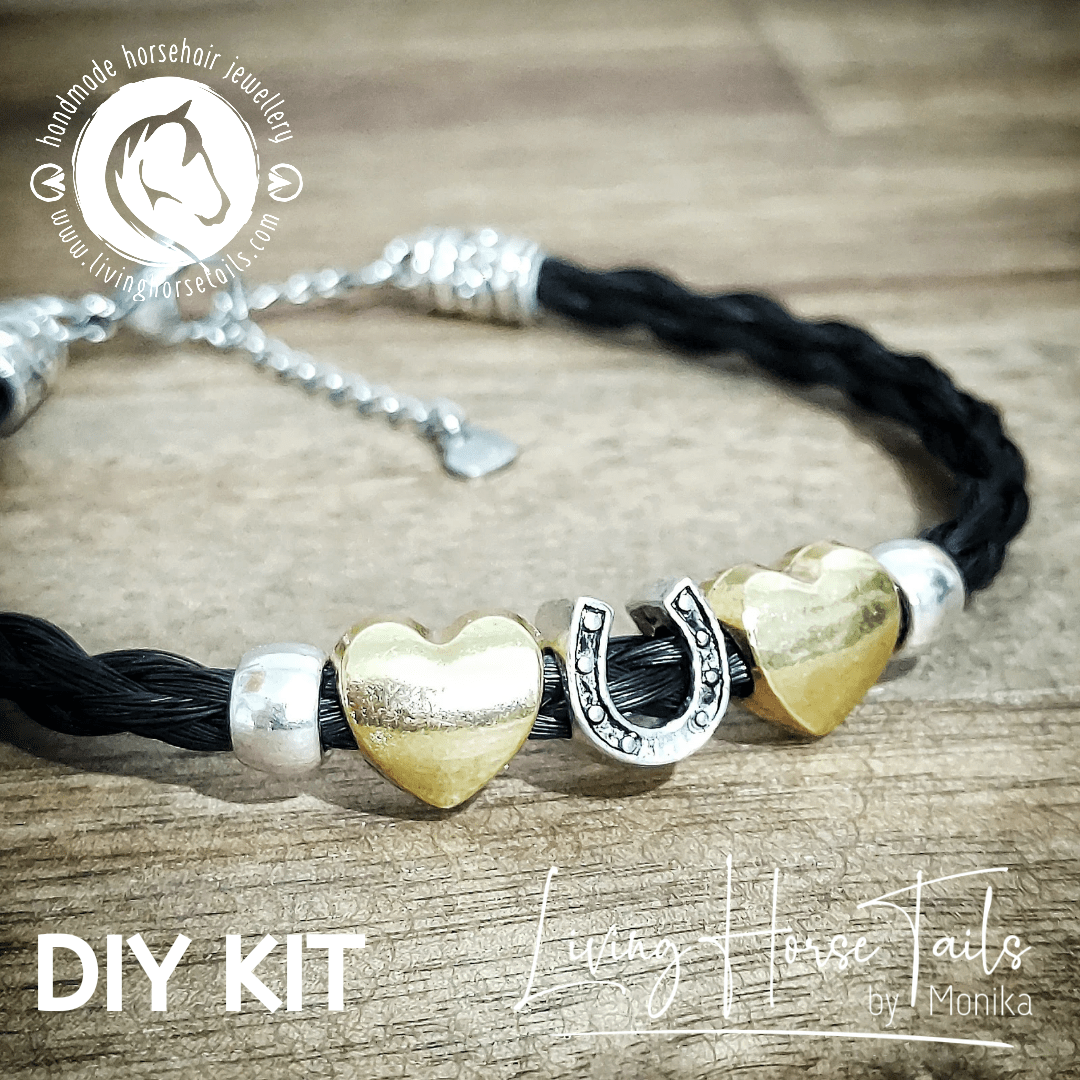This detailed photograph showcases a DIY kit for a necklace called "Living Horse Tales by Monica," displayed on a textured, grayish-brown table. The necklace is elegantly crafted from a robust black cord that is intricately braided into three interwoven strands, resembling leather. The cord culminates in a silver clasp. Adorning the necklace are two gold heart pendants, a central horseshoe charm, and two silver bands, one on each side of the hearts. The text "DIY kit" is prominently placed in white at the lower left corner, while "Living Horse Tales by Monica" is inscribed in loose letters at the lower right. Additionally, the upper left corner is marked with "handmade horsehair jewelry," accompanied by a white circle featuring the silhouette of a horse.